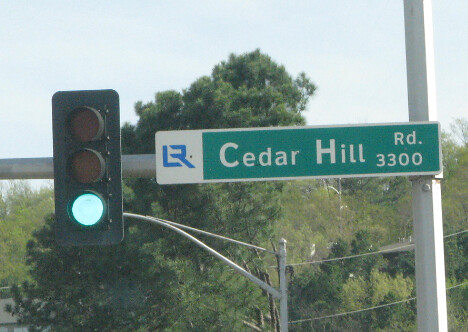In this detailed image, a prominent traffic light and a street sign are depicted in a fairly zoomed-in shot. On the right-hand side, a vertical gray pole with a white outer edge is visible. Mounted on this pole is a rectangular sign displaying "Cedar Hill" and "RD 3300" in white text against a green background. Additionally, there is a white square sign featuring a blue R-shaped logo adjacent to it. Positioned to the left of the pole is a black rectangular traffic light, currently illuminated green. The traffic light is suspended from a horizontal gray rod. Below the traffic light and sign, another pole is visible, surrounded by lush green trees. The upper portion of the image captures a sky transitioning from white to light blue.